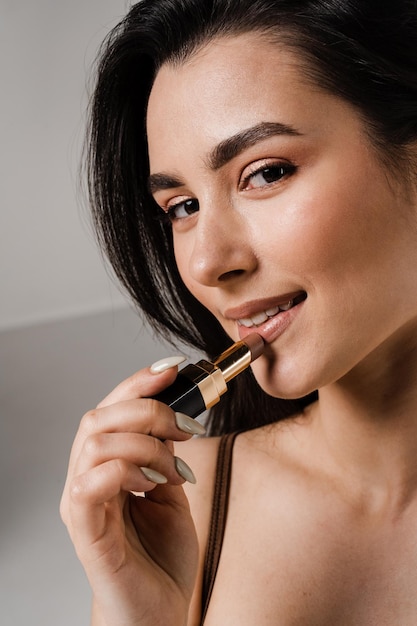The photograph features a female model with an olive complexion, who is artfully applying a brownish mauve lipstick to her lower lip, pressed delicately with a gold and black tube. She has her head turned to the side, looking toward her left, showcasing her thick, dark brown eyebrows, brown eyes, and a half smile. Her long, dark brown hair cascades around her shoulders, just reaching down to her chest but not revealing any nudity. Her right hand, adorned with long, pointed, gray-colored manicured nails, holds the lipstick. The model is dressed in what appears to be a spaghetti strap tank top, indicated by a thin, brown strap visible over her shoulder. The background is a light gray, neutral tone that accentuates the focus on her and the lipstick, creating a professional and well-lit image that might be used for advertising either the model or the lipstick itself.